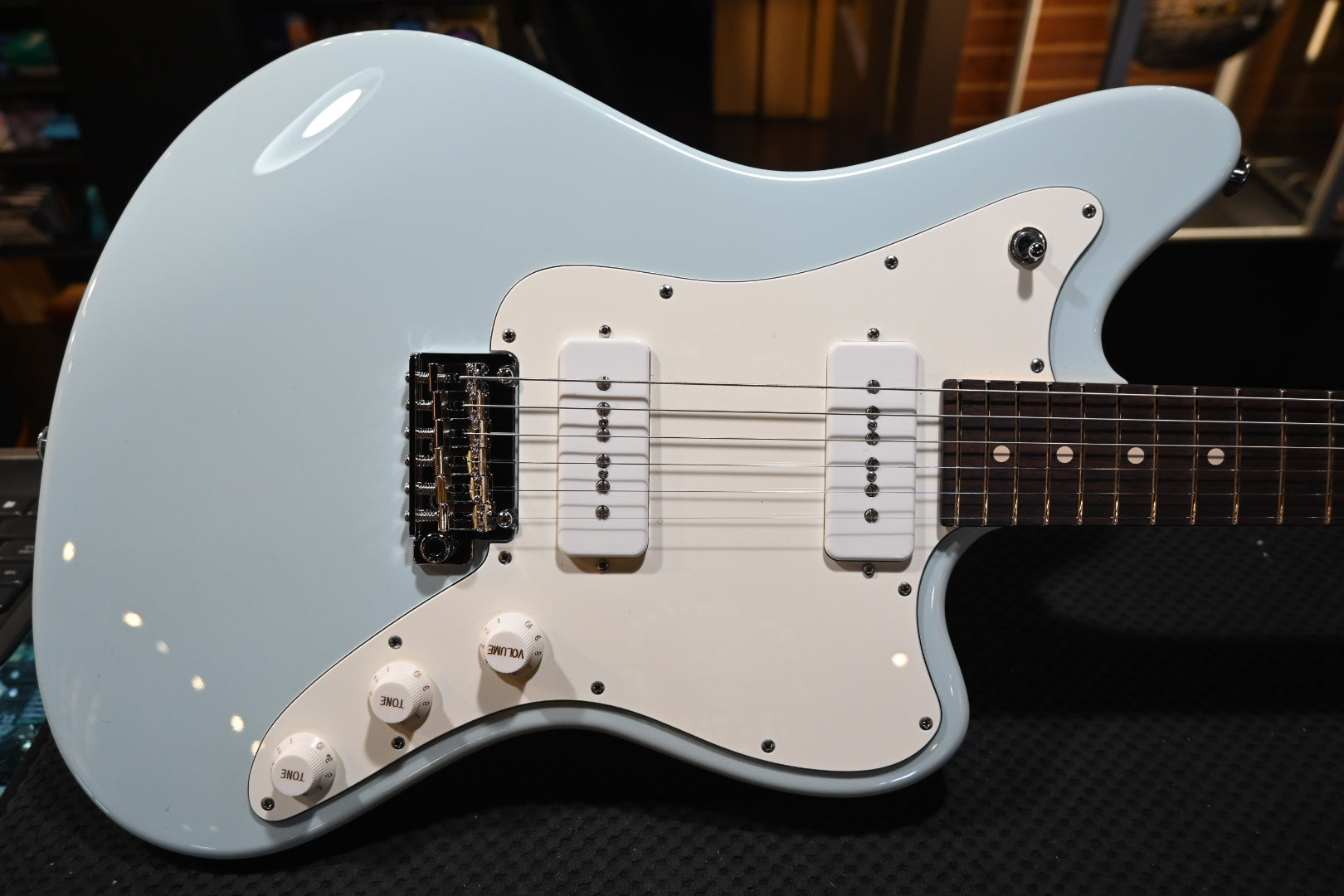The image depicts a light blue and white electric guitar resting on a black surface, possibly padding. The visible part of the guitar includes the complete body and about half of the fretboard, as the image cuts off the upper area with the strings. The guitar features a silver bridge, black pickups, and three control knobs: one for volume and two for tone. There are also white highlights and rivets on the body. In the background, various electronic equipment and what appears to be a glass case or window are visible, suggesting this might be a recording studio or a display in a store or museum. The guitar has six strings and light reflections are noticeable on the left side of its body.